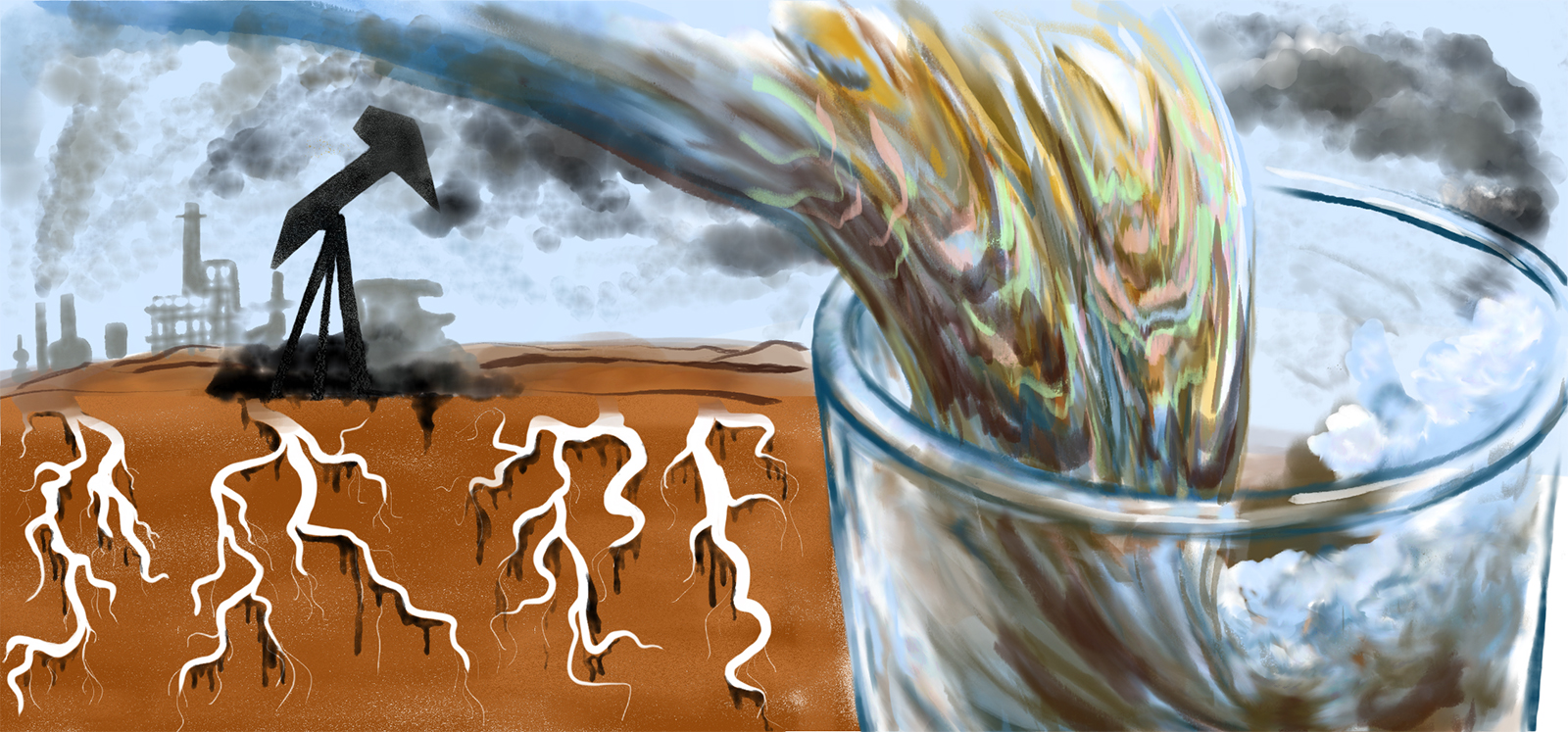This painting showcases a dynamic scene set against a light blue sky with hints of gray smoke. On the left, a black oil rig stands prominently, drilling into the brown earth below. The ground appears fractured with white, lightning-like fissures, possibly indicating sources of oil. Above and behind the oil rig, more shadowy oil rigs emit billowing gray smoke that drifts into the background, blending seamlessly with the sky. To the right, an oversized, clear glass dramatically captures the viewer’s attention. A colorful, swirling liquid, comprised of yellow, brown, and hints of blue, pink, and green, cascades and splashes within the glass, resembling a feather-like shape formed from the smoke. This vivid liquid creates a mesmerizing contrast against the blue background, tying the chaotic industrial elements with an unexpected, beautiful fluidity.